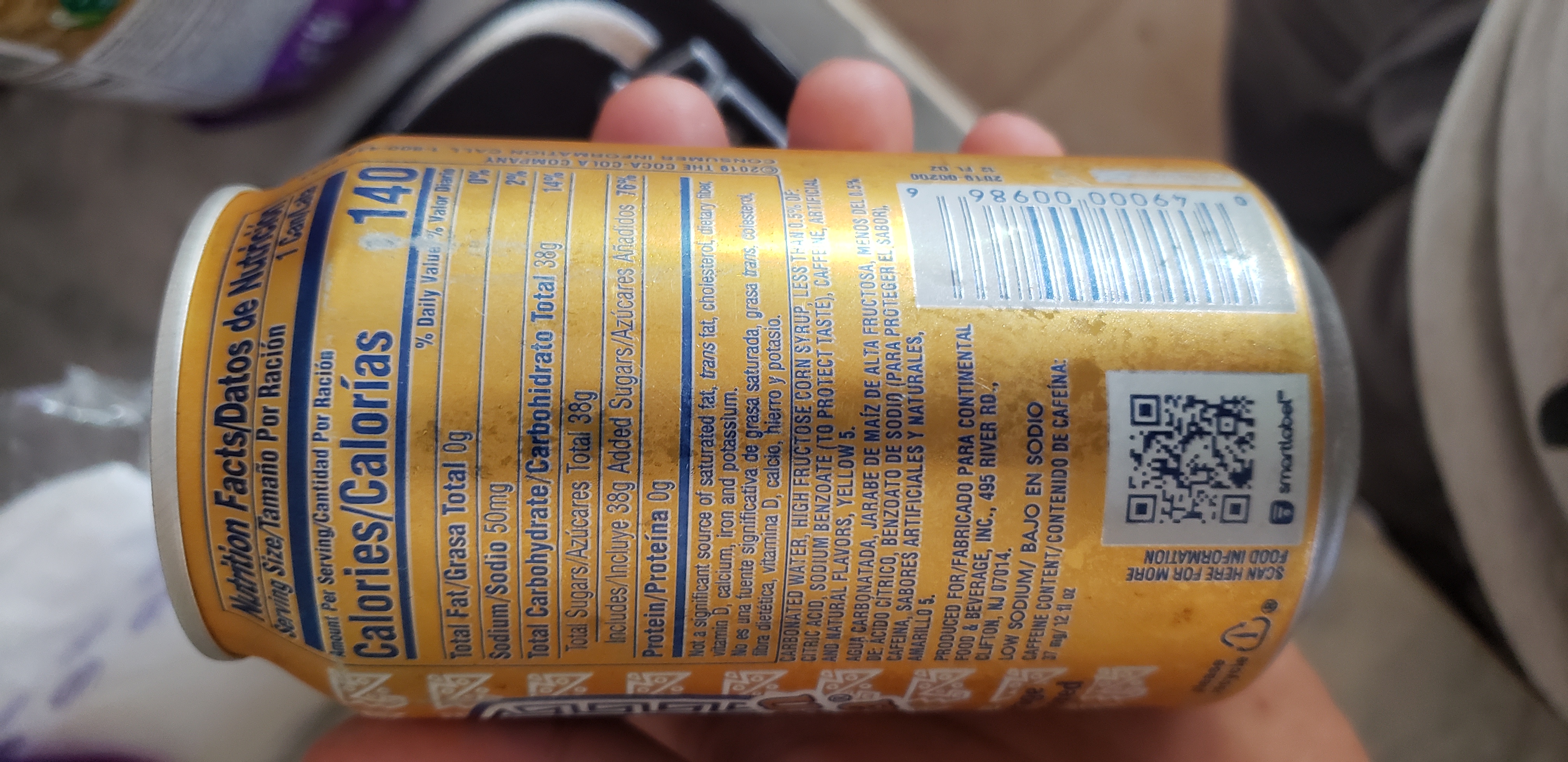The image depicts a person's hand holding a 12-ounce aluminum can of soda, positioned sideways so viewers see the back of the can. The can itself is a golden yellow color with green and blue lettering. Despite the sideways orientation, details from the nutritional label are partially visible, revealing 140 calories. The label, which appears to be written in Spanish, lists various nutritional information including carbohydrates and protein. A scan code is located at the bottom of the can inside a white box, and additional white nutritional information text is present on the side. The camera focuses on the can, making the surrounding environment slightly unclear, but there are hints of metal and tile surfaces beneath the hand holding the soda.